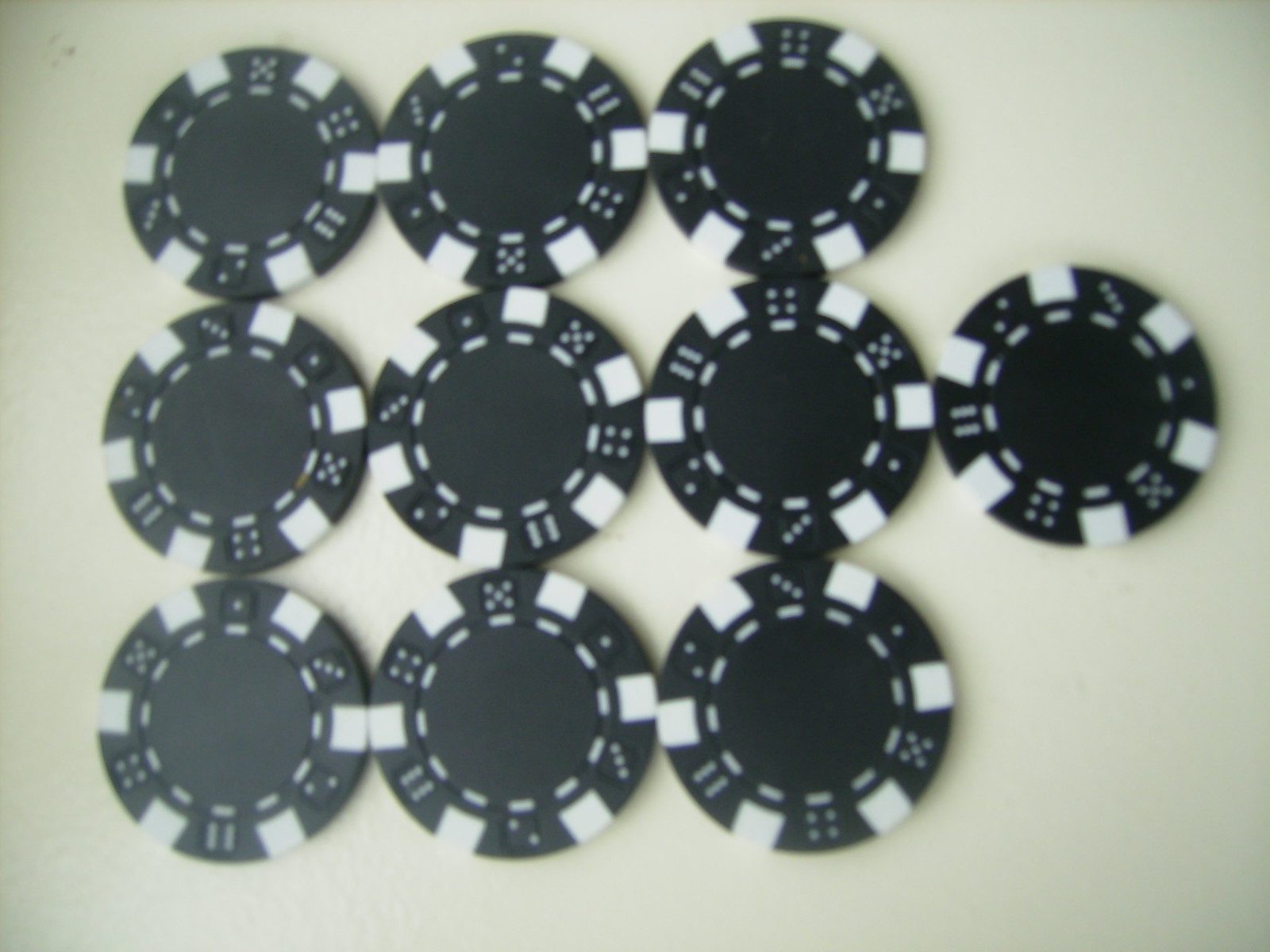This image features a set of 10 intricately designed poker chips arranged on a white surface. Each chip has a uniform design, consisting of a black center encircled by alternating black and white squares. The chips are adorned with faces of a die, depicting the numbers one through six, positioned between the squares. Additionally, a white dotted pattern borders the inner circle of each chip. The chips are organized in three rows: three chips at the top, four in the middle, and three at the bottom. Notably, the photo displays variations in sharpness, with chips on the left-hand side appearing slightly more blurred compared to the more crisply rendered ones in the center. The light source seems to emanate from above, creating minimal shading but noticeable shadows towards the right edge of the image.